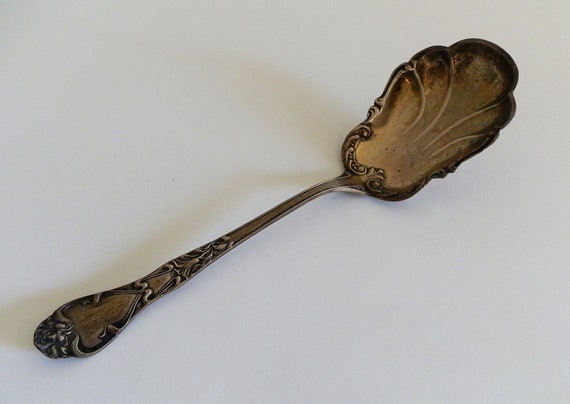This color photograph, taken in landscape orientation, captures an antique serving utensil believed to be from the Victorian era. The utensil, resembling a large spoon, is a dark silver-bronze color, indicating oxidation and perhaps tarnish due to age. The handle, positioned in the lower left corner of the image, is adorned with intricate carvings, including ornamental designs featuring grape-like motifs, swirl patterns, and vine-like elements. The handle is wider at the top and narrows as it nears the scoop. The scoop itself, placed in the upper right corner, is not perfectly round but rather shaped like a flower petal or elliptical with a scalloped edge. It has elaborate decorations within, including veins and fluted shapes, adding to its ornate appearance. The spoon, set against a modern light gray surface, is portrayed in photographic representational realism, emphasizing the detailed craftsmanship and historical essence of the piece.